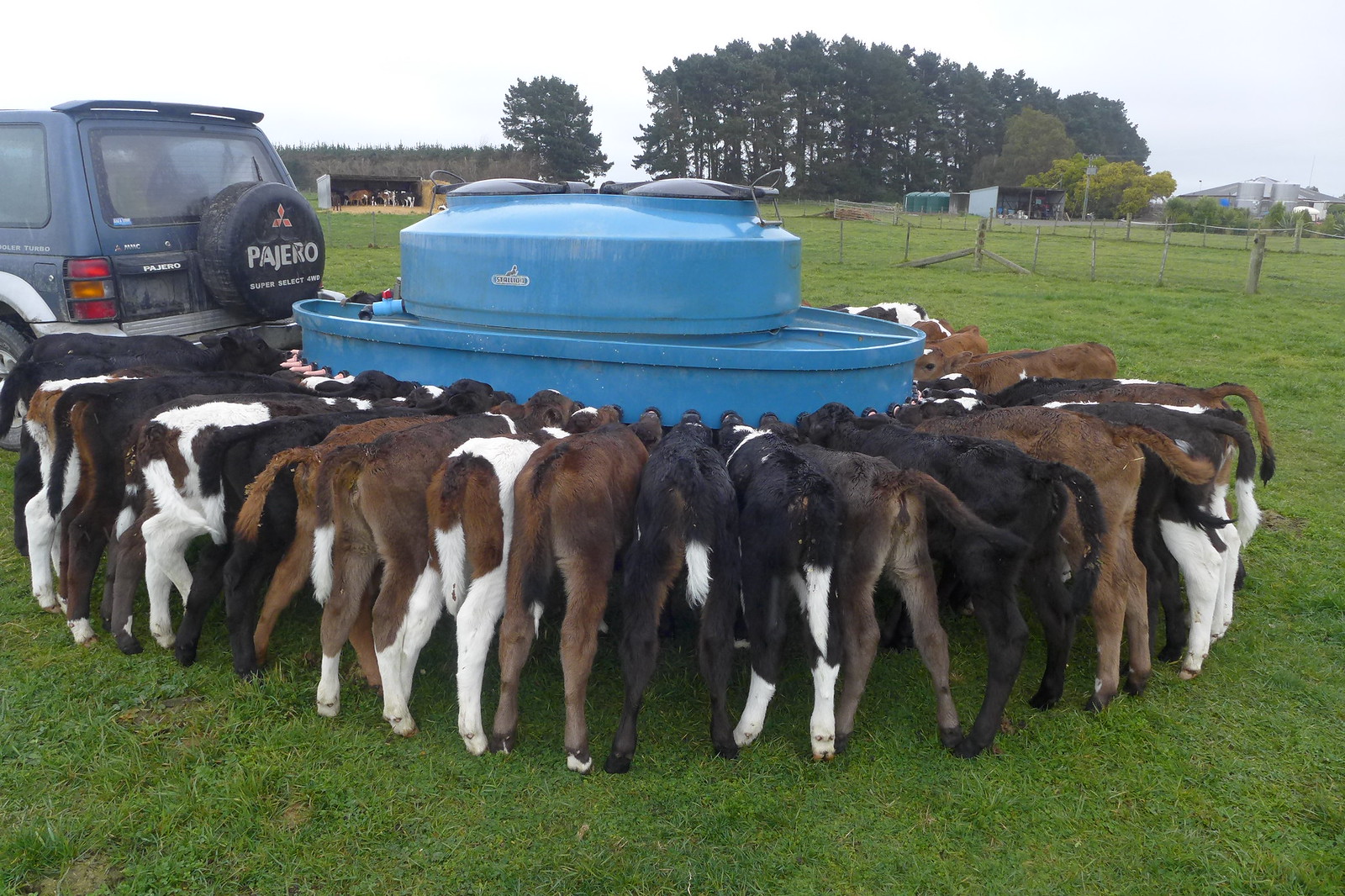The image is a color photograph taken on a farm with low rolling hills covered in green pasture and a small hillock topped with mature trees in the top center. The rest of the foreground features lush green grass, wooden fences, and another hill visible in the upper right. Central to the image is the tail end of a dark blue SUV, which appears to be towing a large blue feeder that looks like a portable feed trough or wading pool with black lids for dispensing feed. Around this feeder, a tightly packed circle of approximately 20 young calves (possibly up to 30, extending beyond the visible area) are gathered, feeding. These calves are a mix of brown, black, white, and spotted colors. Their heads are not visible as they are completely focused on the feeder, and their backs and hind legs face the camera. This pastoral scene showcases the calves clearly congregating around the feed station on a vibrant green pasture.